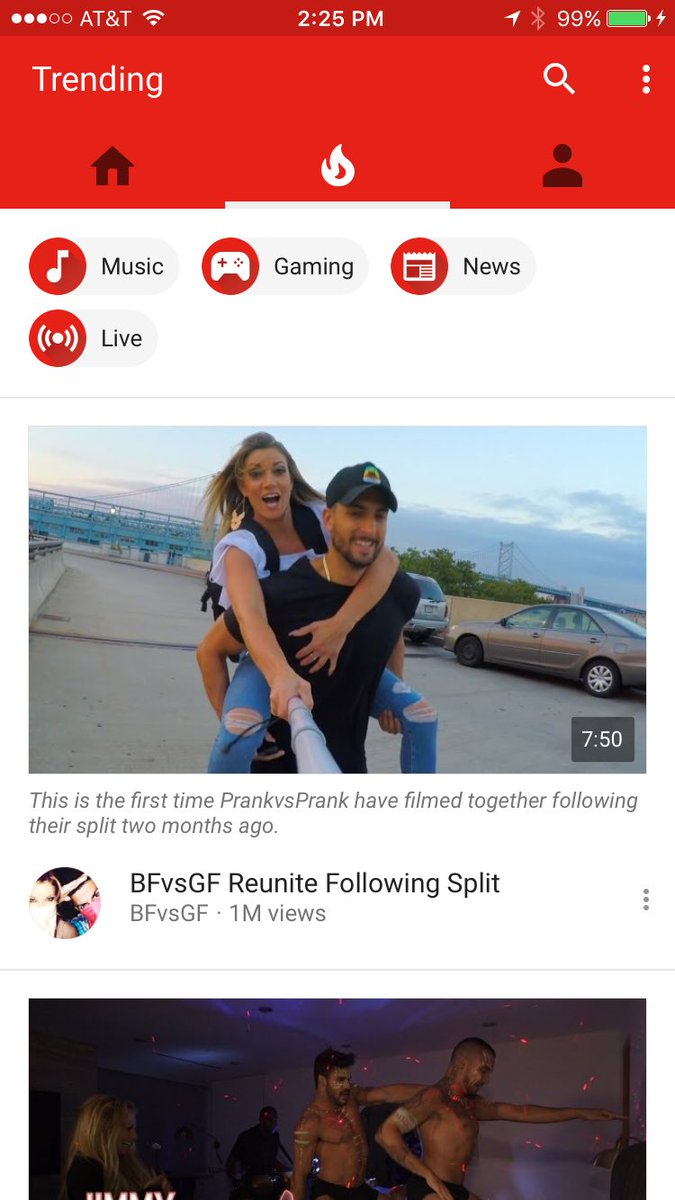The image appears to be a screenshot taken from a mobile or tablet device, though the specific operating system is not identifiable. The device is connected to the AT&T network with three out of five signal bars filled and shows a full Wi-Fi connection. The current time displayed is 2:25 PM. The location sensor is active, while the Bluetooth icon appears grayed out but might still be on. The battery level is at 99% and is currently charging.

At the top of the screen, there is a red bar with white text that reads "Trending." To the right of this text, a white magnifying glass icon is present for search purposes, alongside three vertical dots likely representing additional options.

Below the top bar, there are three navigation icons. The icons include a black house, a white fire symbol (indicating that it is currently selected or highlighted), and a black person silhouette. Beneath these icons, there are additional round, red icons featuring white symbols: a music note for music content, a gaming controller for gaming, a newspaper page for news, and an icon resembling an antenna with parentheses for live content. The user appears to be in the "Videos" section.

The first visible video thumbnail features a white woman wearing a white shirt and blue ripped jeans, appearing excited or shocked while holding a selfie stick. Next to her is a man with a scruffy beard wearing a black shirt and a blue baseball cap. The video is 7 minutes and 50 seconds long and has garnered 1 million views. The video's title indicates it is the first collaboration of "Prank vs. Prank" following their breakup two months ago, titled "BF vs. GF reunite following split."

Below this video thumbnail is a partially visible thumbnail of another video featuring two topless men leaning against a wall, with bandages on their arms, hinting at some other type of video content. The platform appears to be an app or website designed for viewing various types of videos.